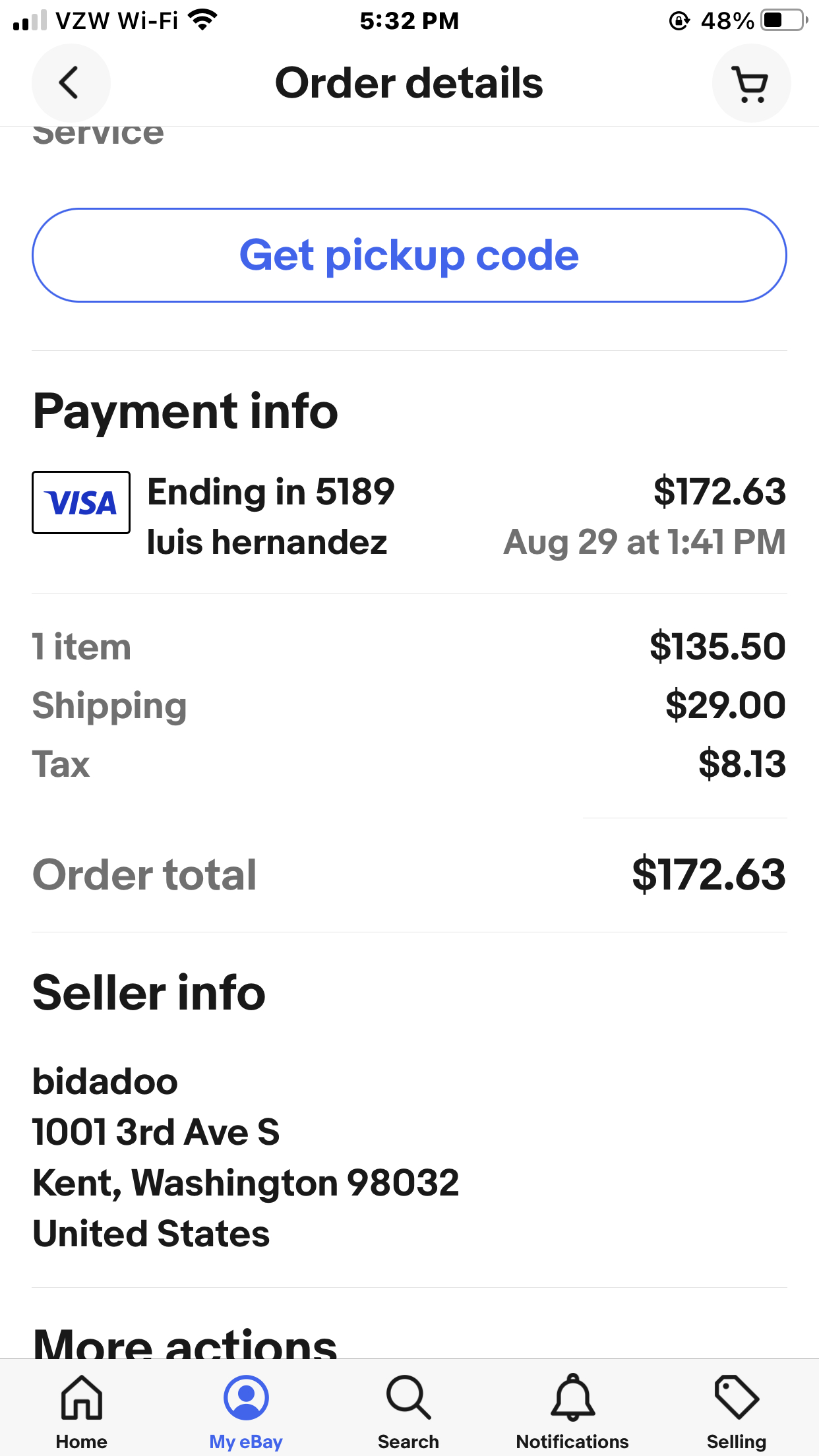This image resembles a screenshot taken from a smartphone. The device's interface elements are visible, including a battery indicator at 48% located in the top-right corner. In the center of the top bar, the time reads 5:32 PM. The top-left corner displays options indicating cellular service strength and Wi-Fi connectivity.

Below the top bar, bold text reads "Order Details," with a back arrow to its left for navigating to the previous screen. On the right side, there's an icon for viewing the shopping cart. Underneath, a button labeled "Get Pickup Code" is housed in a white box with blue text against a similar white background, blending with the rest of the screen.

The "Payment Info" section follows, detailing the payment method: a Visa card ending in 5189, belonging to Luis Hernandez. The total purchase amount is $172.63, itemized as follows: one item priced at $135.50, shipping costs of $29.00, and taxes amounting to $8.00.

Finally, "Seller Info" is prominently displayed at the bottom. The seller's details are listed as Boobadoo, located at 1001 Third Avenue South, Kent, Washington, United States.